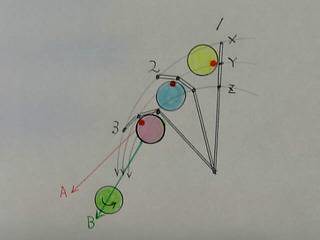This image features an arrangement of interconnected spheres, each distinctly labeled with numbers and letters. The spheres are systematically connected, forming a structured network. The detailed labeling and connections suggest a representation of a molecular structure or a data visualization model. The meticulous design highlights the relationships between each sphere, providing a clear and informative visual summary of the dataset or molecular composition.